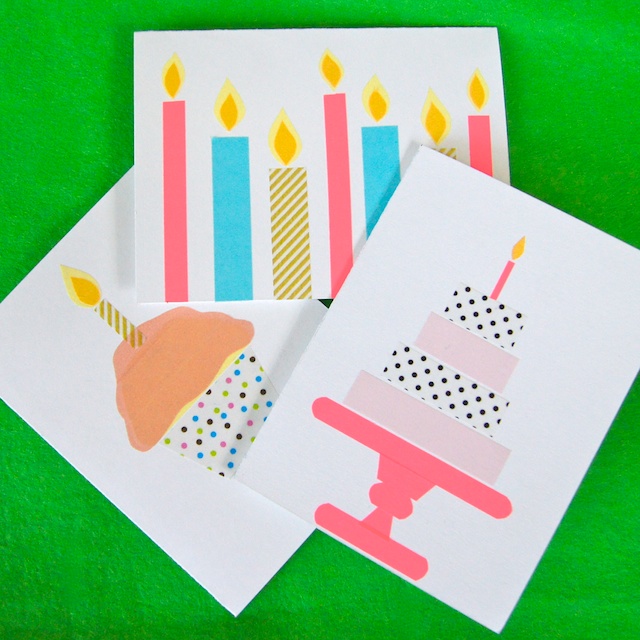This photograph captures a top-down view of three white rectangular papers or cards, neatly arranged on a vibrant green surface. Each card features a distinct birthday-themed illustration. The leftmost card showcases a cupcake adorned with orange-brown frosting, dotted wrapping, and a lit candle. The middle card displays an array of candles in pink, blue, and brown, each candle alight and standing at different heights. The rightmost card depicts a multi-layered cake on a pink table, crowned with a lit candle. The warm yellow flames of the candles create a celebratory essence across all the cards, making them appear as festive birthday invitations or crafts.